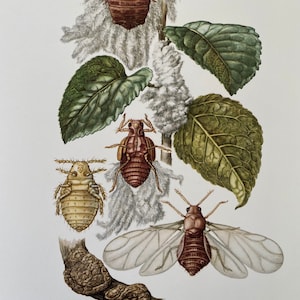This is a detailed illustration depicting a plant stem with three large leaves against a white background. The central stem runs vertically through the image, featuring two green leaves on the right—one dark forest green and the other a lighter lime green—and one leaf on the left showcasing a golden underside. Attached to the plant are four insects with varying colors and textures. Below the lower right leaf, a winged insect appears upside down, displaying its belly and legs. To the left of this winged insect are two more; one has a lustrous coppery-red body, and the other flaunts a shiny gold hue, both showing off their segmented underbellies. Above the top leaf, a partial glimpse of an insect's bottom peeks into the frame. The insects vary in shades from mocha brown to bright yellow. The illustration also includes a white, cottony material along the stem, which might represent a fungus, a plant disease, or a site for egg-laying, adding a layer of biological intrigue to the image.